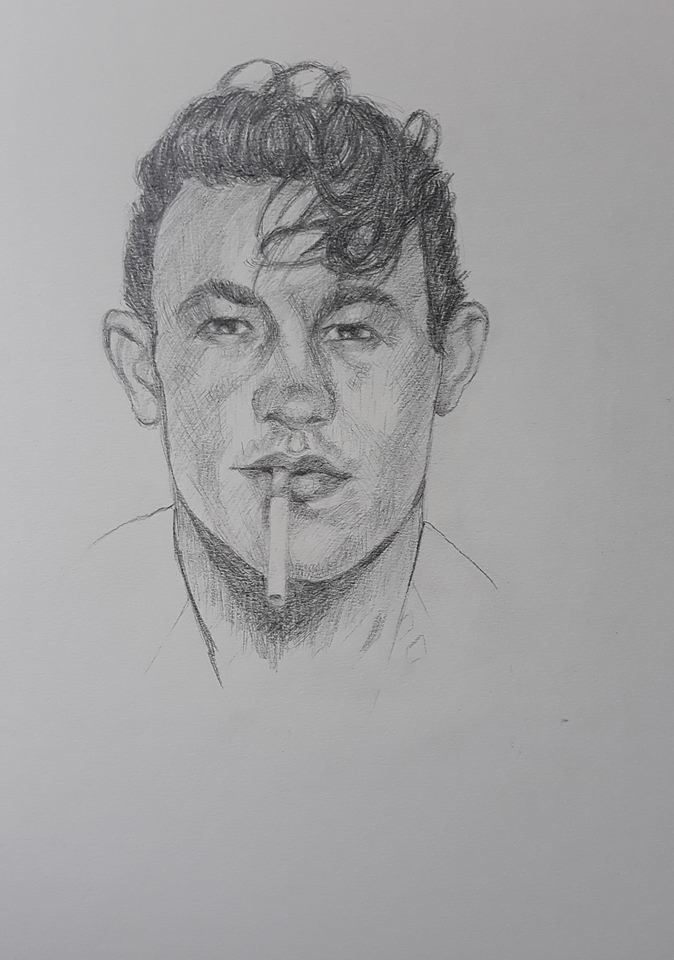The image features a meticulously detailed black and white drawing prominently centered on a white background, devoid of any other elements. At the heart of the image is the head of a person rendered with fine lines and careful shading. The individual's hair is clearly visible, along with their ears, neatly crafted eyebrows, and expressive eyes, which gaze directly forward. The drawing captures the person's distinct facial features, including a well-defined nose and slightly parted lips, from which a cigarette dangles. The depiction extends to reveal part of the person's neck and shoulders, though the rest of the body remains unseen. The stark contrast between the black ink and the white backdrop accentuates the intricate details of the head, giving it a striking presence.